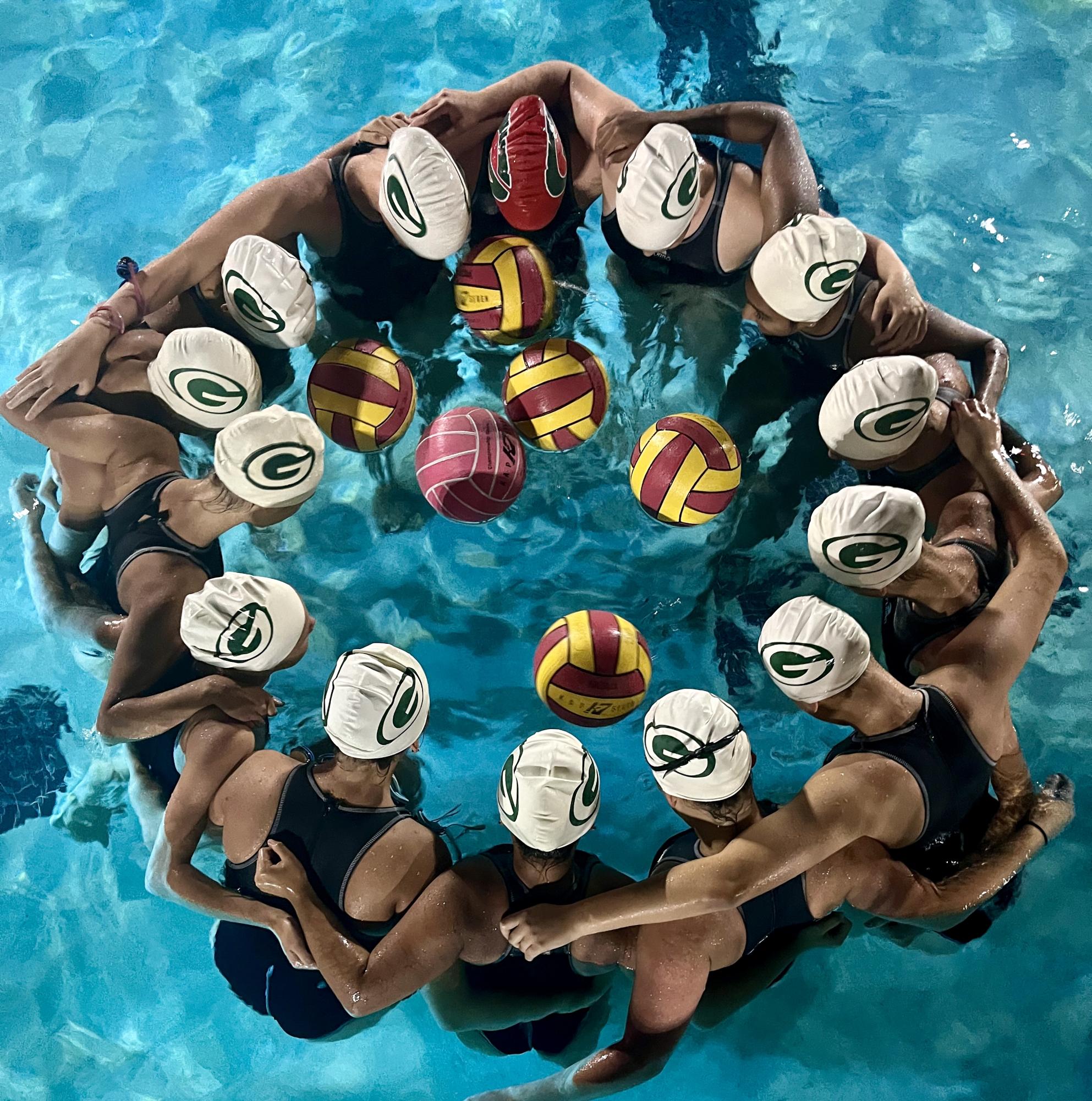The image features a group of swimmers, likely a co-ed or women's volleyball team, huddled together in the center of an indoor pool with sky-blue, rippling water. They form a tight circle with their arms over each other's shoulders and heads bowed, as if psyching themselves up before or after a game. Each swimmer wears a dark navy or black one-piece swimsuit and a white swim cap adorned with a Green Bay Packers "G" logo near the ear area, except for one swimmer who has a red cap with the same logo. In the middle of their huddle, six volleyballs of varying colors float – five have maroon and goldish-yellow sections, while one is completely maroon. The overall atmosphere suggests a moment of camaraderie and team spirit.